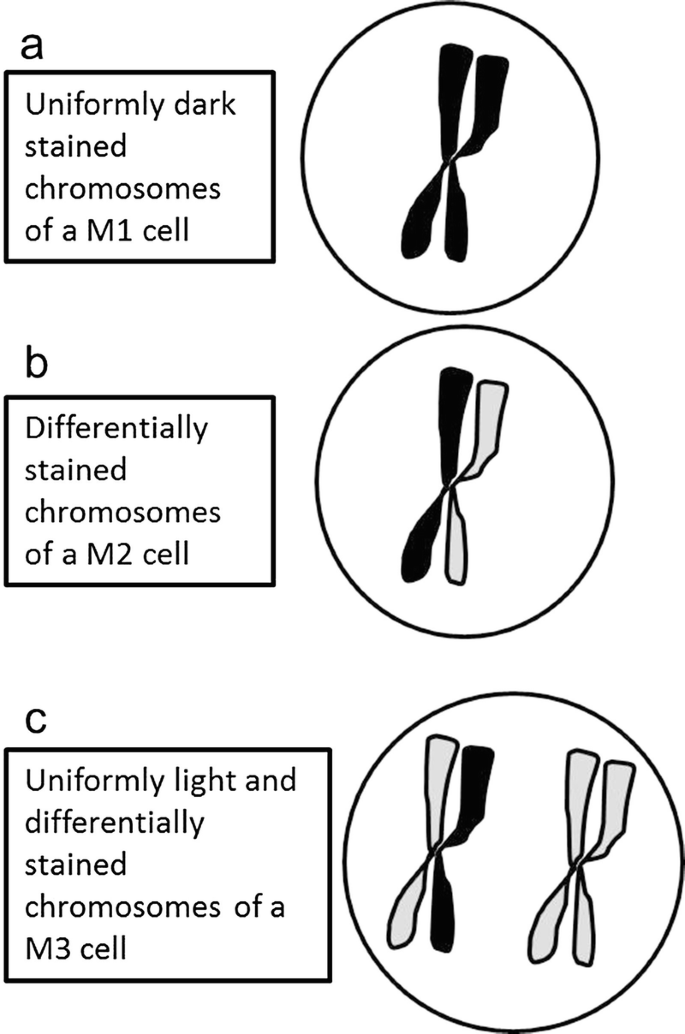The image is a vertically rectangular, simple two-color print piece with a nearly white background. There are three sections labeled A, B, and C, each enclosed within black-bordered squares accompanied by illustrative circles, explaining differentially stained chromosomes for educational purposes. 

Section A features a square labeled "uniformly dark stained chromosomes of a M1 cell," showing a single dark chromosome. Adjacent to it, in a circular illustration, are two black structures crisscrossing to form an X shape. 

Section B is labeled "differentially stained chromosomes of a M2 cell," displaying a chromosome with the right side gray and the left side black. The corresponding circle depicts a similar X-shaped chromosome with a gray right side and black left side. 

Section C contains the label "uniformly light and differentially stained chromosomes of a M3 cell," comprising two X-shaped chromosomes. One is entirely gray, while the other consists of a half black right side and a gray left side.